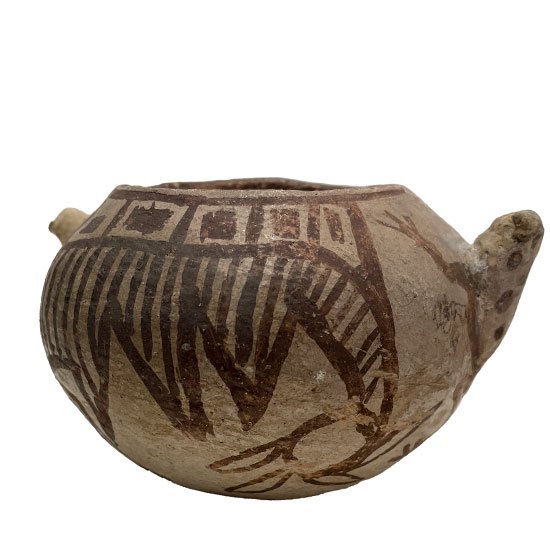This image depicts an ancient, handmade pottery vessel that appears to be of significant historical value, possibly African or Native American. The pottery is tan to brown in color, made of natural clay, indicating considerable age and antiquity. The vessel resembles a pot with an open mouth, without any lid, suggesting it could have been used to transport liquid or other substances. 

The right side of the pot features a spout or an old handle, while the left side has what looks like a broken handle or an ambiguous extension. The pot's surface is adorned with intricate and artistic designs. Prominently, there are squares bordered by white boxes, with triangles extending downward from these squares. The lower portion of the vessel includes a faint pattern that resembles a leaf or branch with leaves. Additionally, the spout or handle on the right side is decorated with brown dots, which might be either decorative elements or stains. 

Notably, the designs are rich yet somewhat ambiguous, featuring symbols and geometric patterns but no text or inscriptions. This ancient vessel, with its deep historical resonance and delicate patterns, stands as a beautiful artifact from a bygone era.